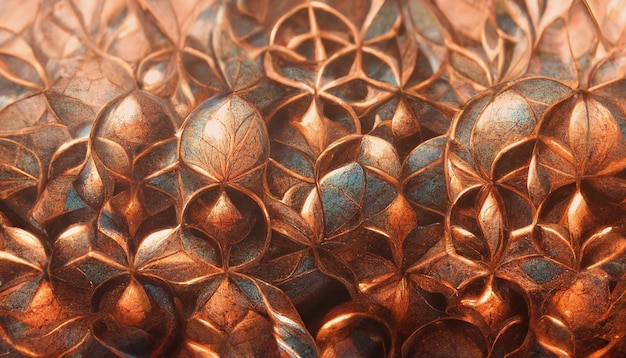This image is a computer-generated illustration in the style of a colored pencil drawing, featuring an intricate, abstract design. It depicts interlaced, gilded leaf-like shapes and circular forms that resemble scales, all rendered in a palette dominated by dark orange, bronze, and copper tones, with hints of pewter, brass, and occasional tarnished spots displaying dark gray and bluish hues. The pattern fills the entire landscape-oriented frame, creating a continuous, repetitive array that evokes a rusted, metallic texture, blending organic and industrial aesthetics.